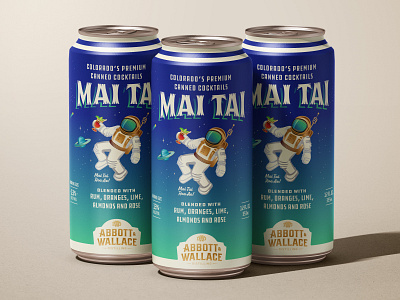This detailed photograph captures three cans of Mai Tai, Colorado's Premium Canned Cocktails, perfectly lined up in front of a white backdrop. The cans are designed with a silver top, followed by a white stripe, a blue stripe, and another white stripe, before transitioning into a blue hue that gradually fades into a greenish color towards the bottom. The very bottom of the can features a silver strip. Dominating the center of the can's design is a white astronaut, depicted floating in space and holding a red drink in his right hand, with planets illustrated in the background. White text across the can prominently states "Mai Tai" and further below in smaller text declares "Colorado's Premium Canned Cocktails." At the bottom, a small emblem with a white background and gold lettering reads "Abbott Palace." The careful lighting casts soft shadows of the cans to the right, enhancing the composition of the image.